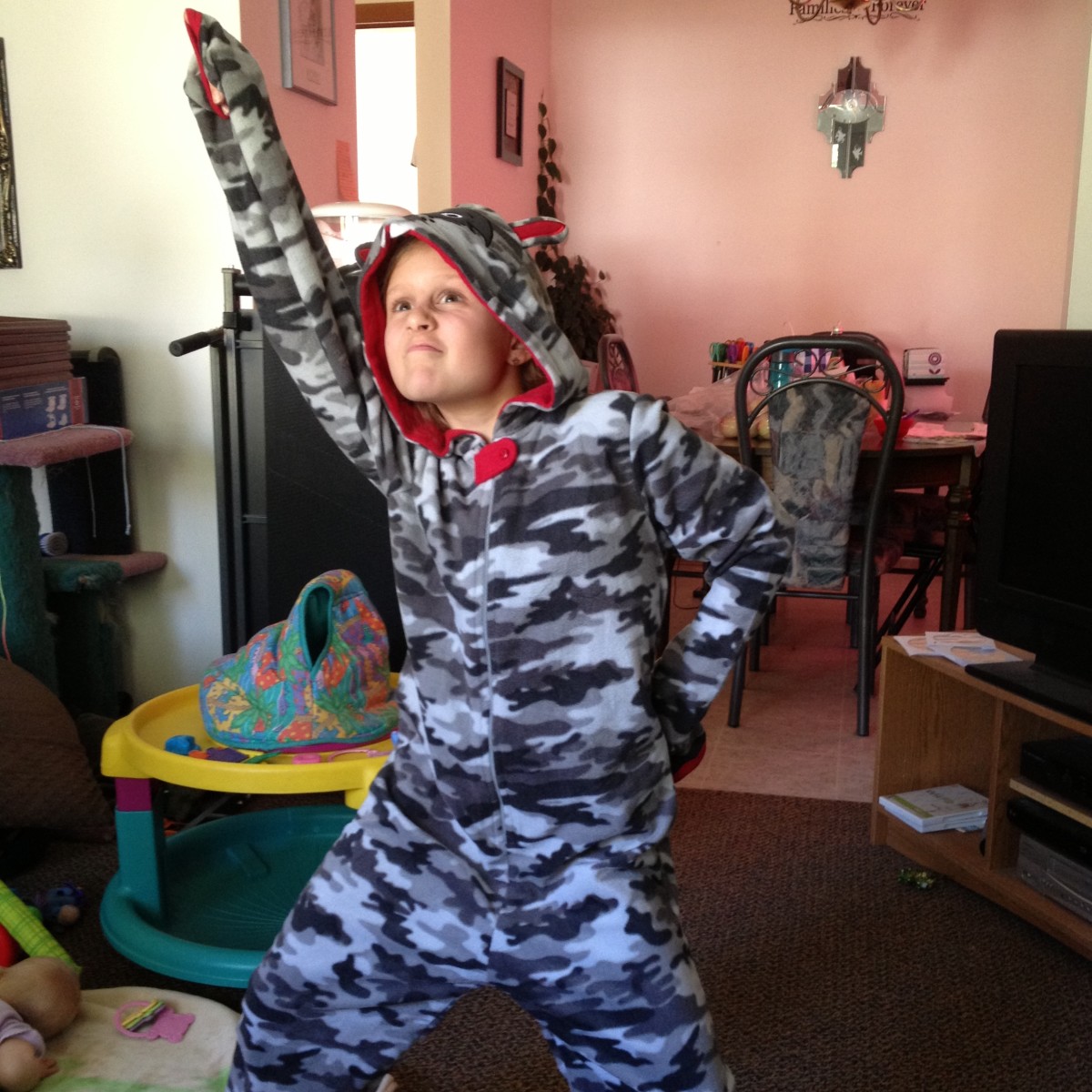The indoor daytime photograph captures a young boy, possibly around nine or ten years old, standing in the center of a room. He is wearing a full-body gray, white, and black camouflage pajama suit with a hood lined in red fabric, featuring little ears on top lined with the same red material. The hood also has a black mask with eyes on top, partially visible. With a mock serious expression, flared nostrils, and left hand on his hip, the boy points upward off-screen with his right arm, though his hand remains inside the sleeve, making it unseen. He stands with legs extended to both sides, bracing his chin with a posture of confidence. The room's background shows a kitchen area with pink walls, a brown area carpet, a dining table with black chairs, and other cluttered elements like a baby walker with a yellow top and a teal base draped with a bag and toys. Additionally, a low entertainment credenza in brown grained MDF wood with a large screen television sits nearby, along with various undetermined items scattered around.